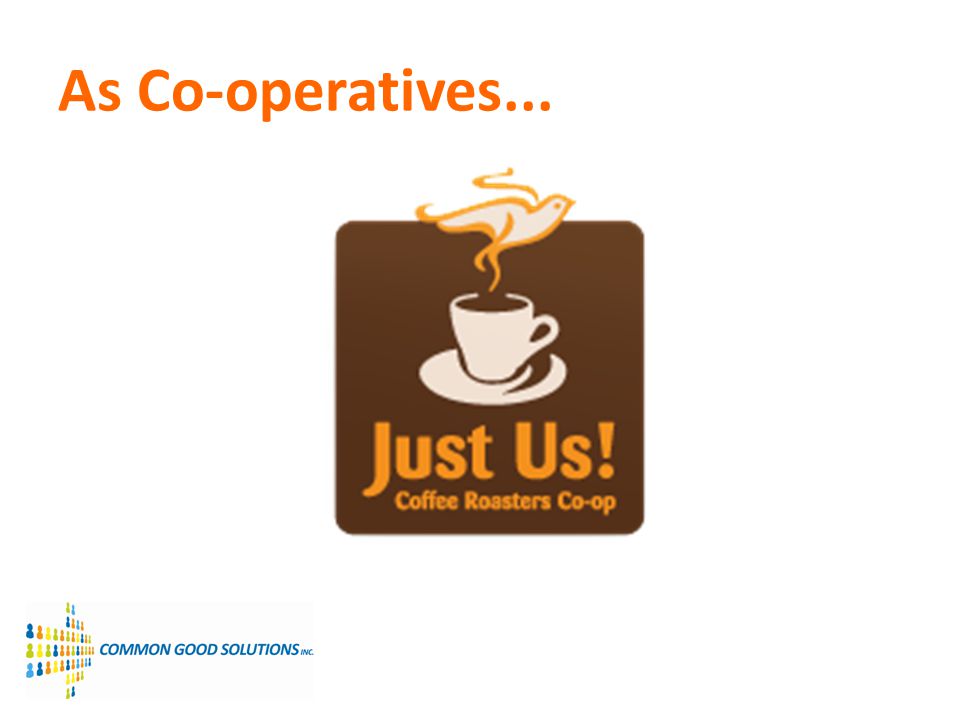The image features a predominantly white background with the title "As Co-operatives..." written in orange letters at the top. At the center, there is a brown square with rounded corners containing a white coffee cup on a saucer. Rising from the coffee cup is steam that forms the shape of a bird outlined in light orange. Below this coffee cup logo, the text reads "Just Us! Coffee Roasters Co-op" in orange. Towards the bottom left of the image, the words "Common Good Solutions, Inc." are visible next to a right-pointing arrow composed of iconographic figures in various colors including blue, yellow, orange, and green.